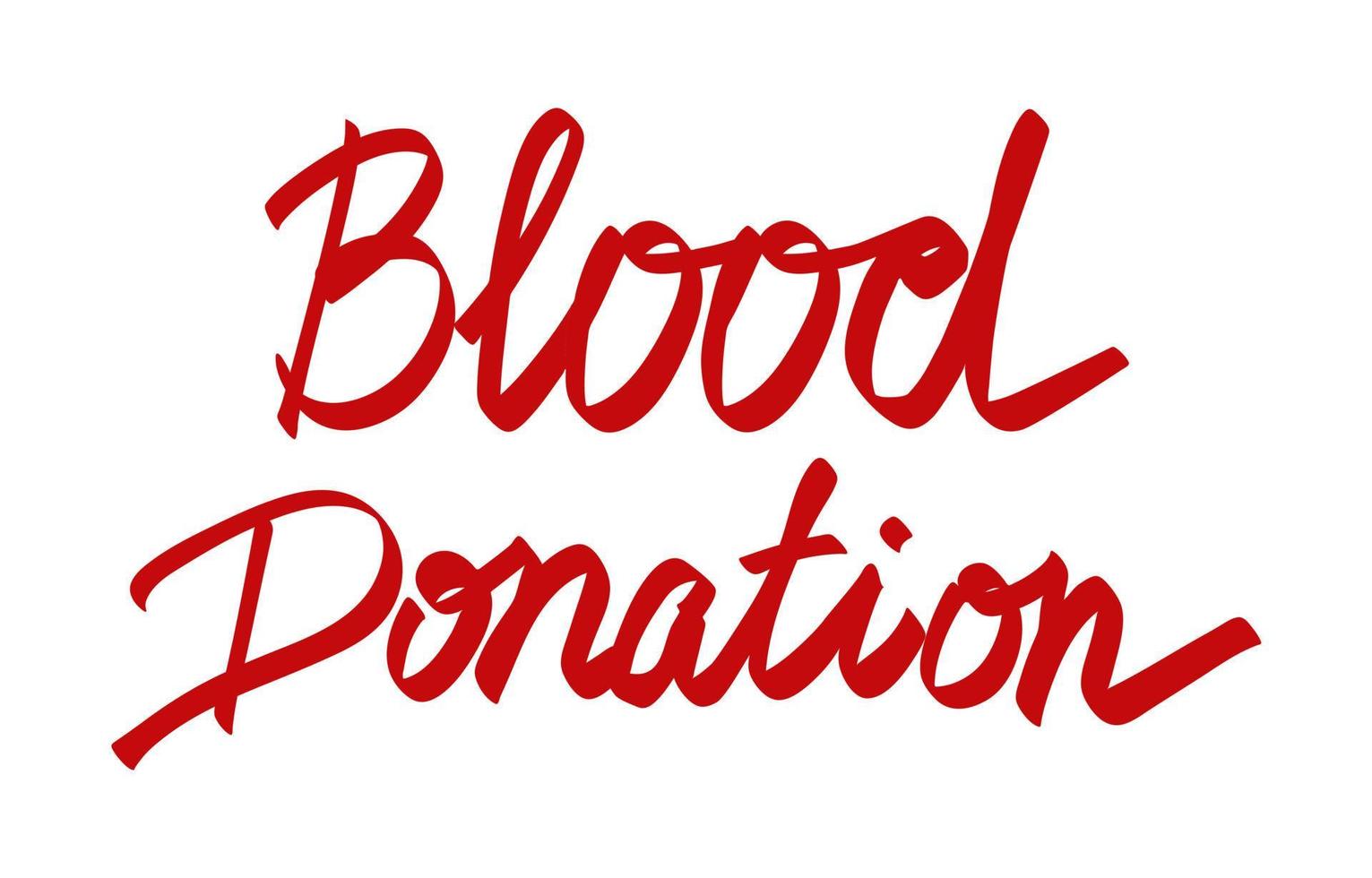The image features a stark, solid white background that occupies the entire surface area. Centered in the middle of this background are two red cursive words, written in what appears to be a flat-tipped permanent marker. The first word, "Blood," is on the top line with a capital 'B' followed by lowercase letters. Directly below it, the second word, "Donation," also starts with a capital 'D' and continues in lowercase. The cursive script has a hand-drawn quality, with thicker parts where the loops occur and thinner sections at the bends, creating a dynamic, swirling effect. The text is slightly arched, adding a subtle curvature to the composition.